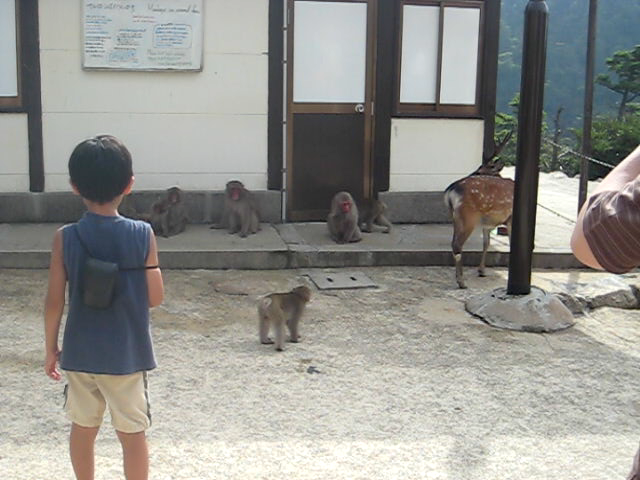In this outdoor daytime scene, a young boy, around seven to nine years old, is seen from the back, wearing a sleeveless blue tank top and khaki shorts. He appears to have a small shoulder strap that might be holding a container for a camera. The boy is standing on a dirt or gravel surface, gazing at a group of small monkeys, possibly macaques or baby baboons, characterized by their pink faces and light gray bodies. Most of these monkeys are sitting on a small porch of a white building with a wood-frame door and windows shaded by white blinds. There's also a whiteboard with writing that is too far away to read. Nearby, on the ground, another monkey is visible alongside a young, spotted deer with skinny legs—a brown body with white spots and black marking near its tail. The scene also includes the elbow of an adult, possibly the boy’s father, on the right side of the image. In the upper right corner, tall jungle-like trees can be seen in the distance, indicating a valley or forested area, adding to the picturesque and sunny ambiance, evidenced by the shadows cast on the ground.